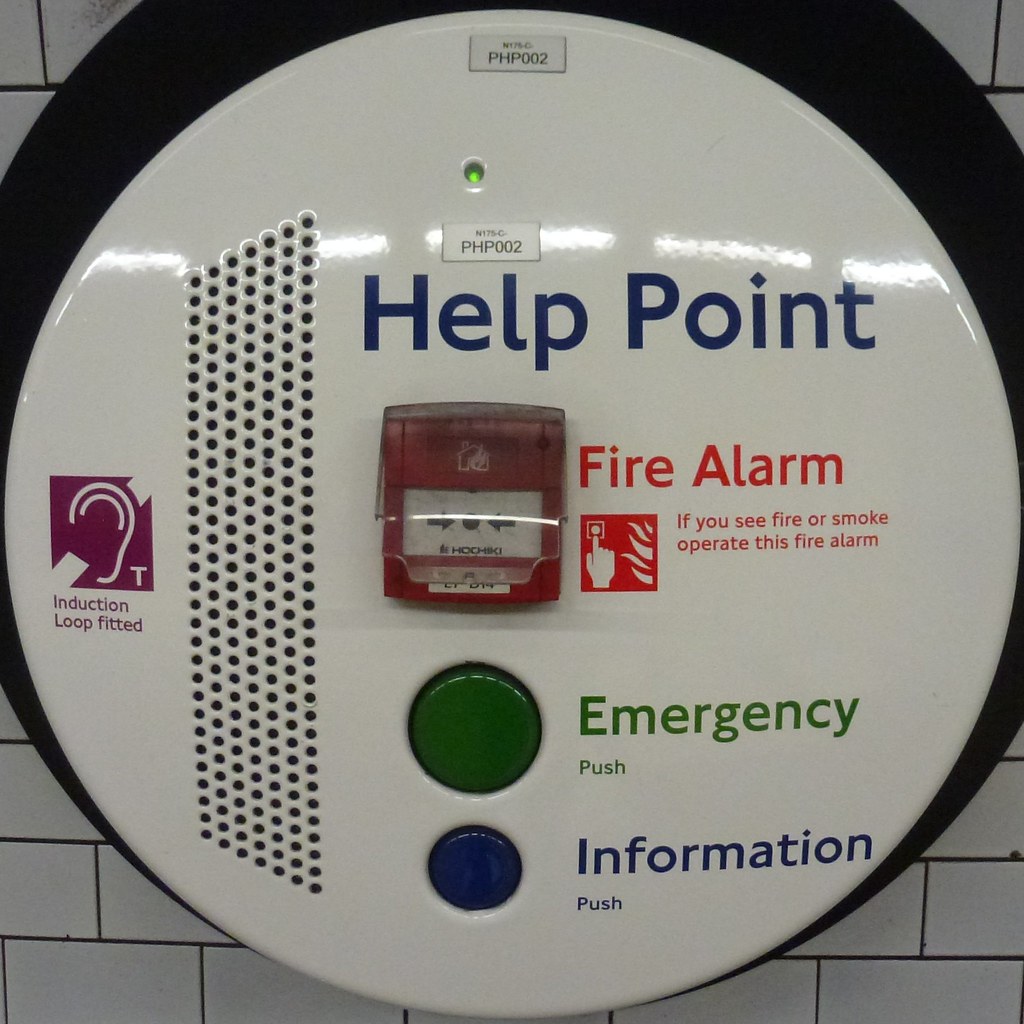The image captures a detailed view of a white, glossy fire alarm mounted on a ceramic brick-shaped, white-tiled wall. The alarm itself is encased in a white, circular station, known as a "Help Point," highlighted by the dark blue text at the top. Surrounding the help point is a black round mounting. This Help Point features various functional areas: on the left-hand side, there's a vertical grid of holes forming a vent, and a purple square beside it with a white ear icon and the text "Induction Loop Fitted." 

Below the Help Point text, there is a prominent red fire alarm indication area. This red square includes the instruction: "If you see fire or smoke, operate this fire alarm," accompanied by an illustration of a hand pressing a button. Just beneath this, a large green button is labeled "Emergency Push," and right below it, a smaller blue button says "Information Push."

Additional markings include a green-lit indicator at the top and two labels that read "BHP002" positioned above the "Help Point" text and at the very top of the device. The image is very zoomed in, allowing detailed visibility of these elements against the tiled backdrop.